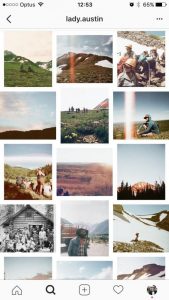**Caption:**

A collection of 12-15 photos captures various outdoor adventures, albeit in unclear quality. The topmost image bears the title "Lady Austin." The photos showcase diverse landscapes and activities: a snow-covered mountain possibly near a ski resort, hikers on a desert trail, a lush green mountain, and a brown-hued mountain reflecting autumnal tones beneath a cloudy sky. Among these, a black and white image stands out, depicting about 15 individuals gathered outside a rustic cabin, hinting at its vintage nature. Another blurred photo features a man wearing a helmet, though the specifics of his activity remain indistinct.